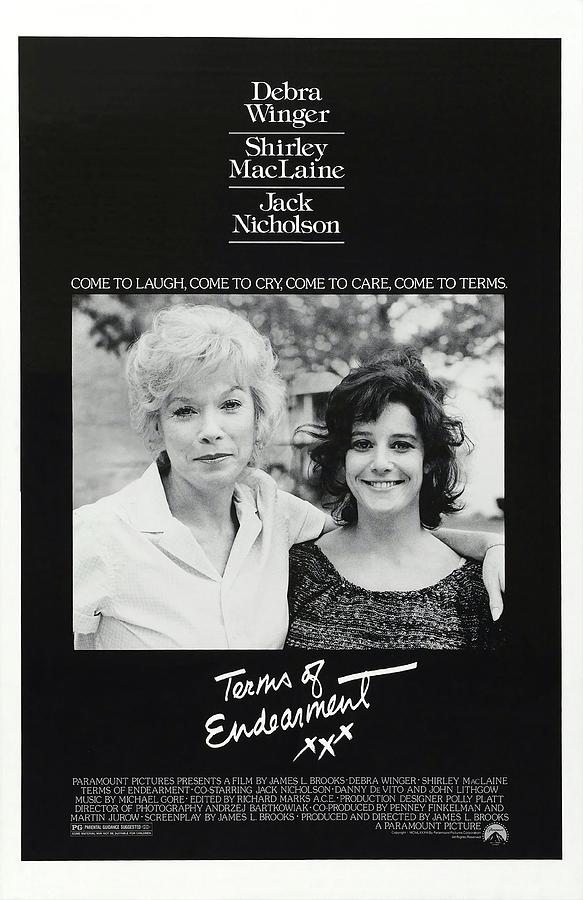The promotional poster for the movie “Terms of Endearment” features a black background with the names of the main actors prominently displayed at the top in white letters: Debra Winger, Shirley MacLaine, and Jack Nicholson, each name separated by a gray line. Below the names, in smaller white text, the tagline reads, "Come to laugh, come to cry, come to care, come to terms." The central image on the poster shows Shirley MacLaine on the left, wearing a white button-up shirt with a collar and light blonde hair, smiling with her arm around Debra Winger, who stands slightly shorter with dark shoulder-length hair. Underneath the picture, the movie title "Terms of Endearment" is written in cursive. The overall background of the poster is black and white, with additional production details listed below the title.